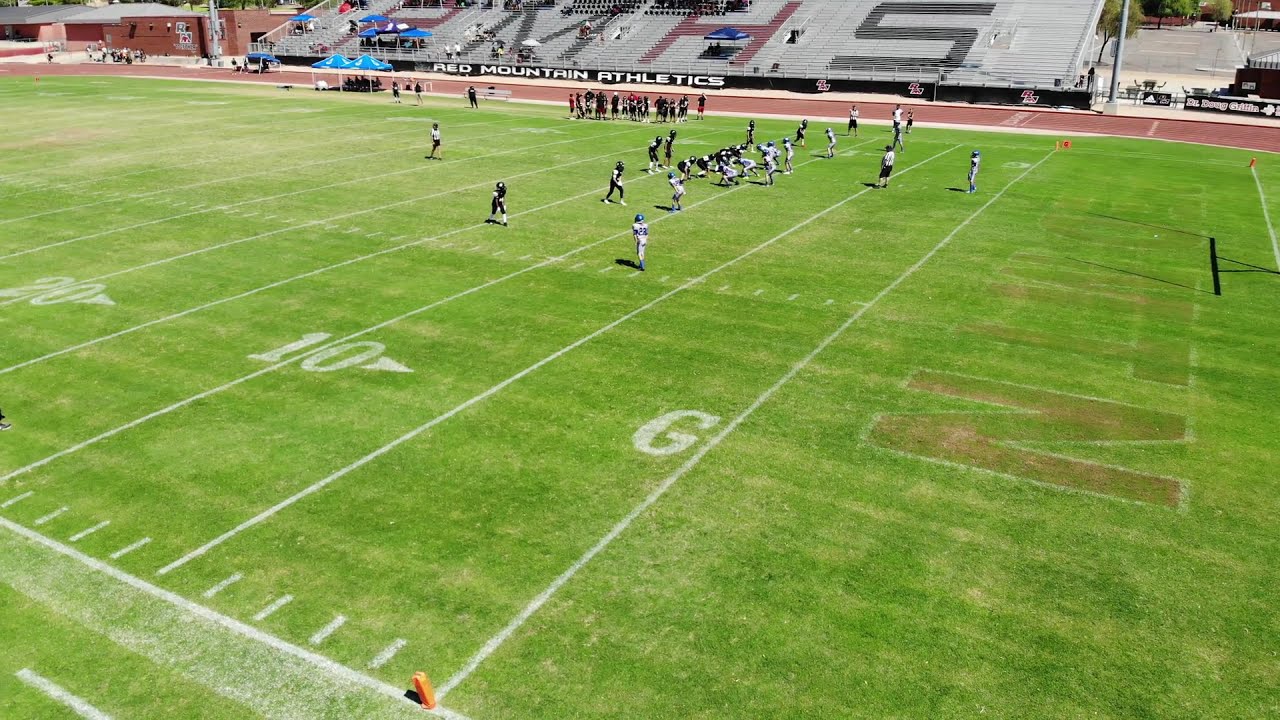An aerial view captures the vibrant scene at Red Mountain High School's football stadium during what appears to be a competitive game, rather than practice. The bright green grass field, marked with crisp white yard lines, stretches out from the end zone, with the ball situated near the 11-yard line. On the field, two teams are in action; the players in white and blue uniforms face off against those in black and yellow. A referee is positioned around the 25-yard line, overseeing the gameplay.

Adjacent to the field, the sideline hosts bench players and two small tents, likely for scorekeeping and game management. Spectators are scattered across the bleachers, under which "Red Mountain Athletics" is displayed in white text on a fence. "RMHS" is prominently painted on the bleachers, signifying Red Mountain High School. Additionally, a brown building stands to the left of the bleachers, with people gathered in front. In the corner of the track that encircles the field, a group of onlookers intently watches the game. The entire scene is bathed in sunlight, highlighting the lively atmosphere of this high school football event.